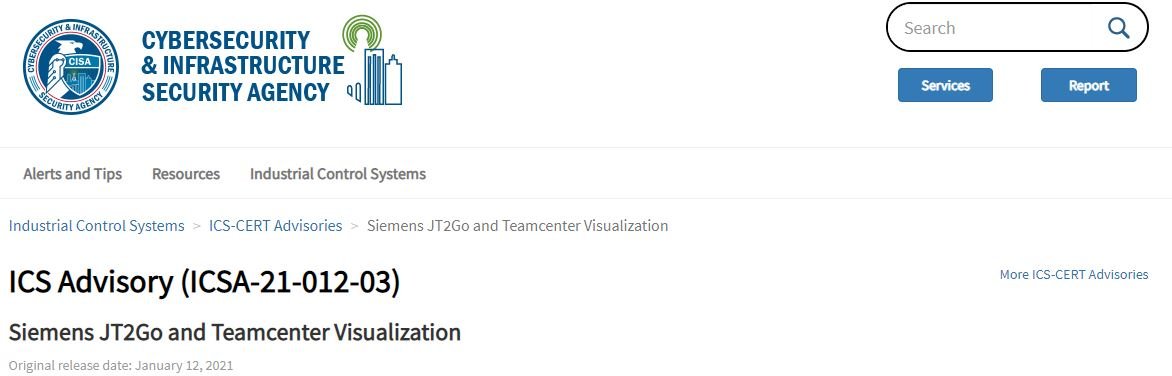In this image, we are viewing a detailed screenshot set against a pristine white background. 

In the upper left corner, there is a medallion-type icon featuring a white eagle at its center. Encircling the eagle, the text reads "Cybersecurity and Infrastructure Security Agency" in blue. Directly to the right of this icon, bold blue text prominently displays "Cybersecurity and Infrastructure Security Agency." 

Towards the upper right, there is an illustrated graphic of a city building, which adds a visual element to the composition. Below these headings, a list of categories is displayed in black text: "Alerts and Tips, Resources, Industrial Control Systems." 

Further underneath, in lighter blue text, the section reads "Industrial Control Systems ICS CERT Advisories Siemens JT to Go and Teamcenter Visualization." 

Then, in large, bold black text, the advisory number "ICS Advisory ICSA-21-012-03" is noted. Following this, the text reiterates in smaller black text, "Siemens JT to Go and Teamcenter Visualization." This detailed arrangement effectively communicates the critical information related to cybersecurity advisories and resources.